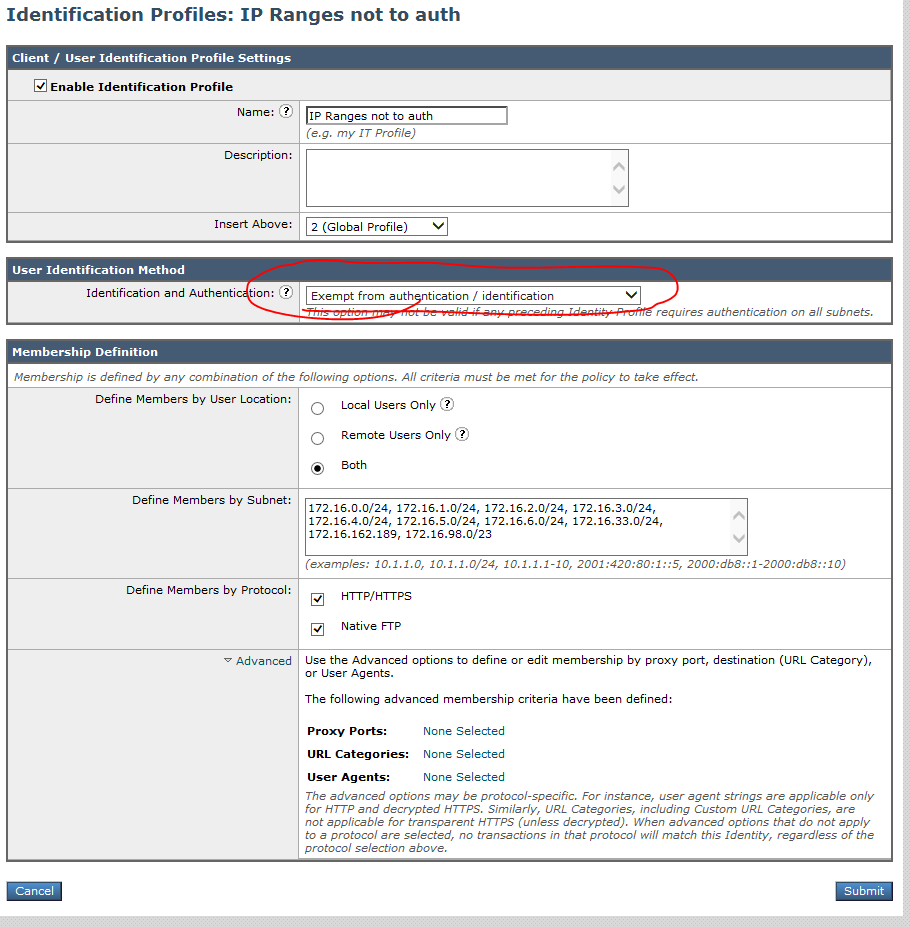This image is a detailed screenshot of a website settings page. 

At the top, there is an empty text box labeled "Global Profile," accompanied by a check mark and a down arrow for selection options.

Below this is a section highlighted with a blue heading titled "User Identification Method." Within this section, there is a label for "Identification and Authentication," which is currently set to "Exempt from Authentication/Identification" indicated by a down arrow. This specific setting is emphasized with a red hand-drawn circle around it.

Further below is the "Membership Definition" section. This section elaborates that membership is defined by meeting several criteria. The following options are presented:

1. **Define members by user location:**
   - Local users only
   - Remote users only
   - Both (Selected)

2. **Define members by subnet:**
   - A text box listing several IP ranges, with the first entry being "172.16.0.0/24."

3. **Define members by protocol:**
   - HTTP/HTTPS (Selected)
   - Native FTP (Selected)

Next, there is another blue header labeled "Advanced." This section provides options to further define membership by proxy port, destination URL category, or user agents. However, all advanced membership criteria in this screenshot are marked as "None Selected."

At the bottom of the page, under a section described as "fine print," there are additional options and information that are not fully visible in the screenshot.

Finally, outside of the main content area of this webpage, there are two prominent buttons: "Cancel" and "Submit," allowing the user to either discard or save the changes made to this settings page.